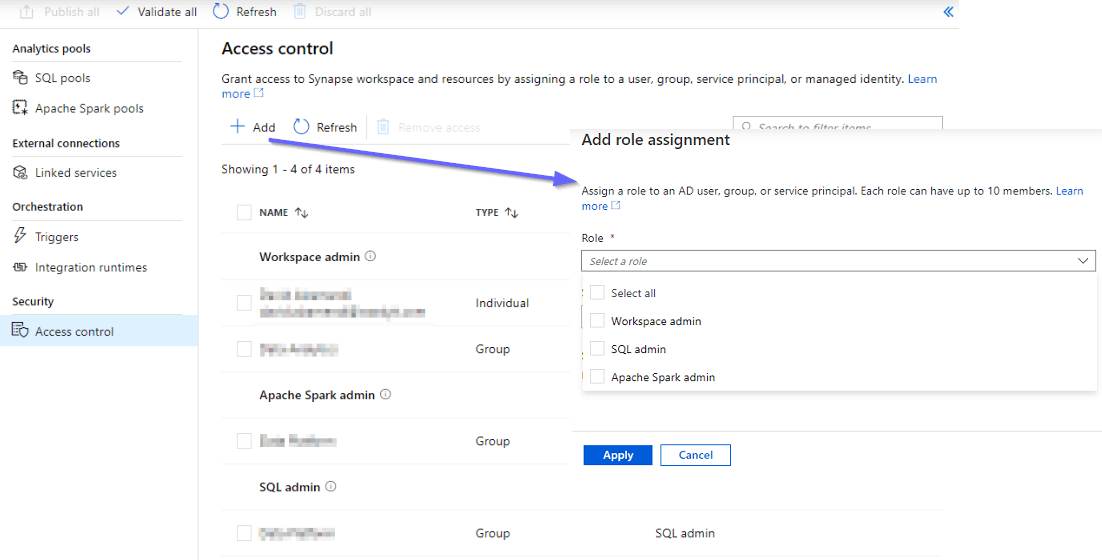This image displays an admin panel interface specifically focused on access control management within a data analytics platform. At the top of the interface, there is a horizontal menu bar featuring several action options: "Publish All," "Validate All" (with a check mark indicating it is currently active), "Refresh," and "Discard All."

On the left side of the interface, there's a vertical navigation menu listing several categories associated with database and integration management: "Analytics Pool," "SQL Pools," "Apache Spark Pools," "External Connections," "Linked Services," "Orchestration," "Triggers," "Integration Runtime," "Security," and "Access Controls." The "Access Controls" category is highlighted in blue, indicating it is currently selected.

To the right, the "Access Controls" section is displayed, which allows the user to grant access to the Synapse Workspace and its resources by assigning various roles to user groups. This section includes controls for "Service Principal," "Managed Identity," options to "Learn More," "Add," and "Refresh." There are visible role assignments, showing one of four entries involving names, types (such as "Workspace Admin" with the type "Individual" and several entries grayed or pixelated out, identified as "Group" roles for "Apache Spark Admin" and "SQL Admin").

Additionally, there are selectable options on the right side that allow the user to "Assign a role to an AD (Active Directory) user group or service principal," with guidelines indicating that each role can accommodate up to ten members. This section also includes a drop-down menu for selecting roles, with available choices being "Workspace Admin," "SQL Admin," and "Apache Spark Admin," all of which are currently unchecked. At the bottom, the user has "Apply" and "Cancel" buttons to finalize or discard the changes. A purple arrow highlights a section pointing towards a text that provides further instructions on role assignment.